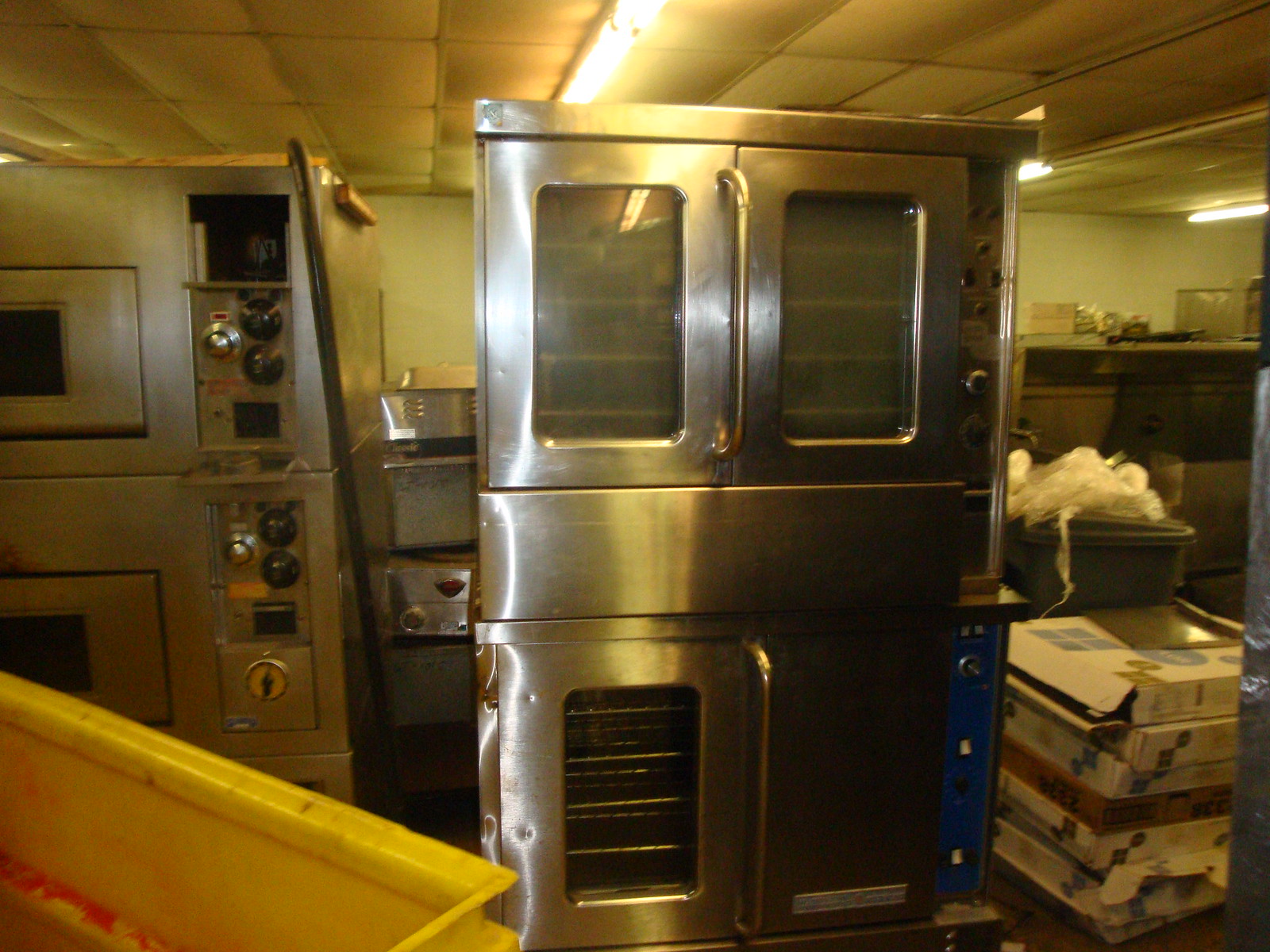This image captures a bustling and well-used industrial kitchen, tinged with a warm yellow light characteristic of indoor illumination. Gleaming silver appliances dominate the space, each exhibiting a dual-tiered structure. Prominently in the foreground, a large, well-worn yellow tub rests on the left-hand side, its scars and scratches testament to frequent use. Adjacent to the appliances, a stack of cardboard boxes, predominantly white with an occasional brown one, suggests they've either been used for deliveries or holding supplies. To the right, hints of a black trash bin peek out from behind the boxes, partially covered with plastic. The kitchen is dotted with various stainless steel ovens and warmers, identifiable by their dual-door configurations with glass sections and multiple control knobs located to the right of each unit. The appliances, polished but industrial, reflect a space designed for heavy-duty culinary tasks. Overhead, dirty ceiling panels mar the otherwise functional aesthetic, contributing to the impression of a hardworking commercial environment. Shelves line the left side of the image, adding to the utilitarian decor, while a white wall provides a stark contrast to the metallic sheen of the equipment.